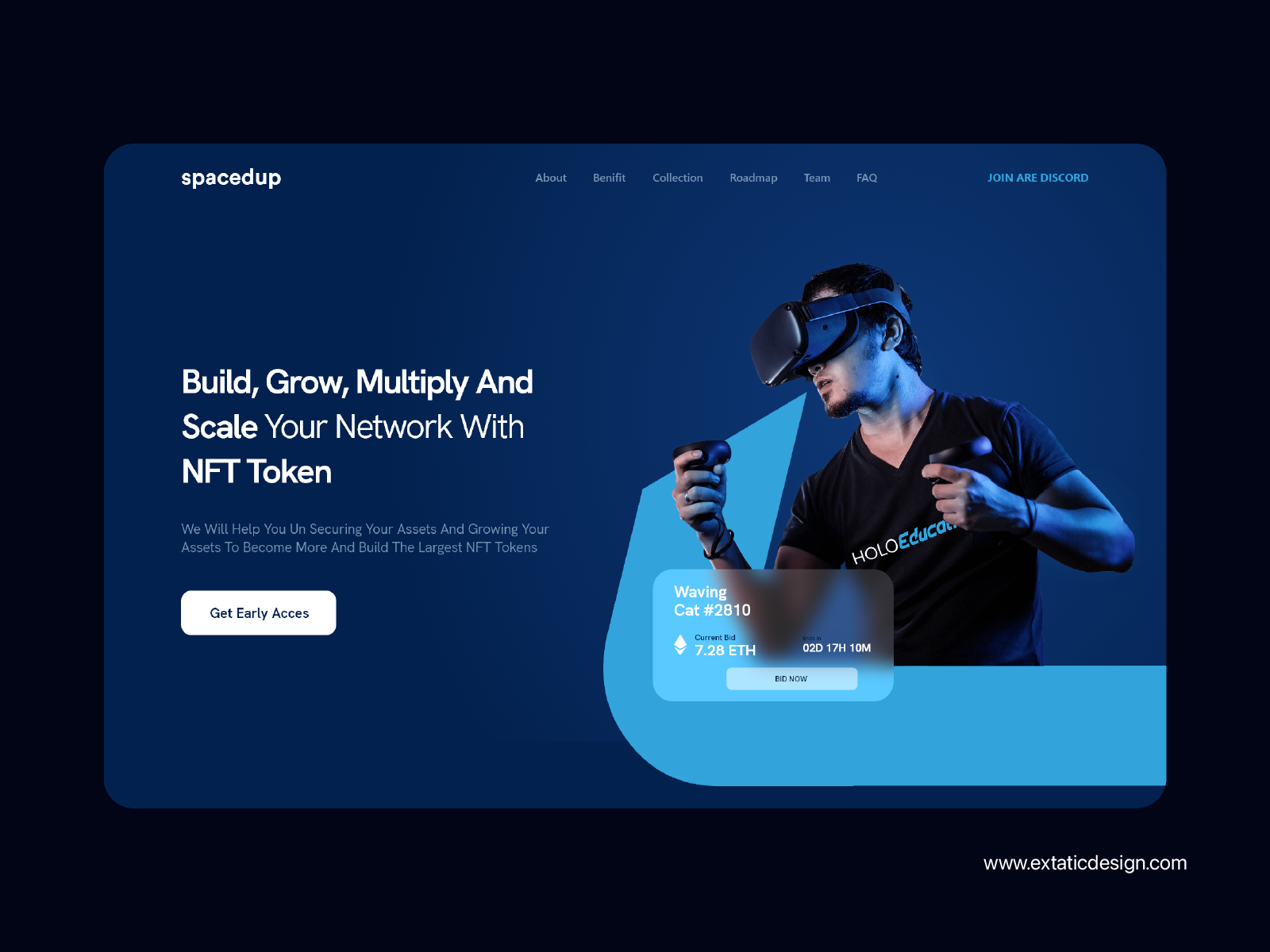The image features the homepage of a website named "Spaced Up," which appears to be a virtual reality (VR) headset company. The background of the webpage is a vibrant blue. The central message displayed prominently reads: "Build, grow, multiply, and scale your network with NFT tokens." The site offers the opportunity for users to gain early access to their services, suggesting a sense of exclusivity and excitement. However, a glaring error is present in their call to action - "Join our Discord" is misspelled as "Join are Discord," using the incorrect form of the word "R". This simple yet significant mistake casts doubt on the professionalism and reliability of Spaced Up, potentially deterring users concerned about the company's attention to detail and legitimacy.